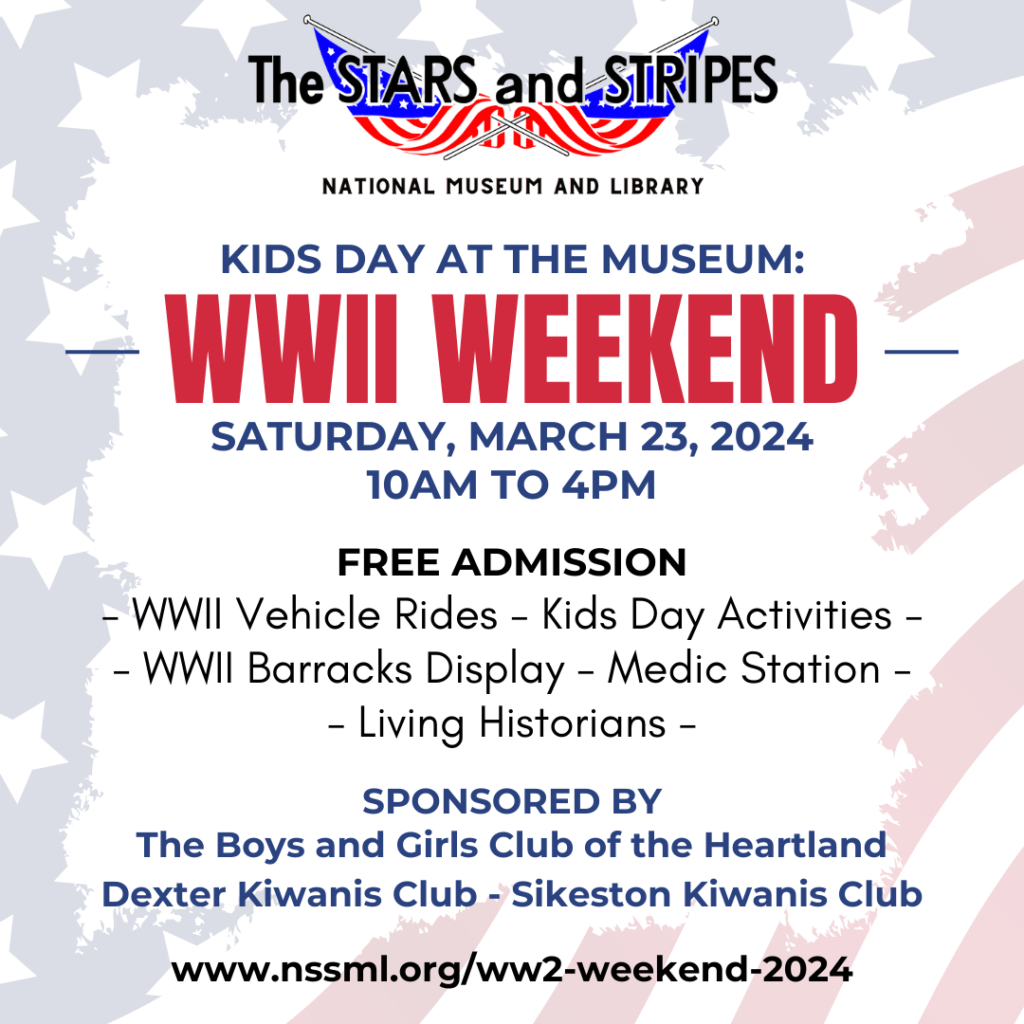This advertisement poster features a white sheet of paper with a large, transparent watermark of the American flag covering the entire background. At the top, the logo for the Stars and Stripes National Museum and Library is displayed, accompanied by two slightly angled red, white, and blue American flags. The main event, "Kids Day at the Museum: World War II Weekend," is prominently announced in navy and red fonts, scheduled for Saturday, March 23rd, 2024, from 10 a.m. to 4 p.m. The poster highlights activities including World War II vehicle rides, Kids Day activities, a World War II barracks display, a medic station, and living historians, all with the benefit of free admission. The event is sponsored by the Boys and Girls Club of the Heartland, Dexter Kiwanis Club, and Sykes and Kiwanis Club. At the bottom of the poster, there's a website for more information: www.rinsml.org/WWIIweekend2024.